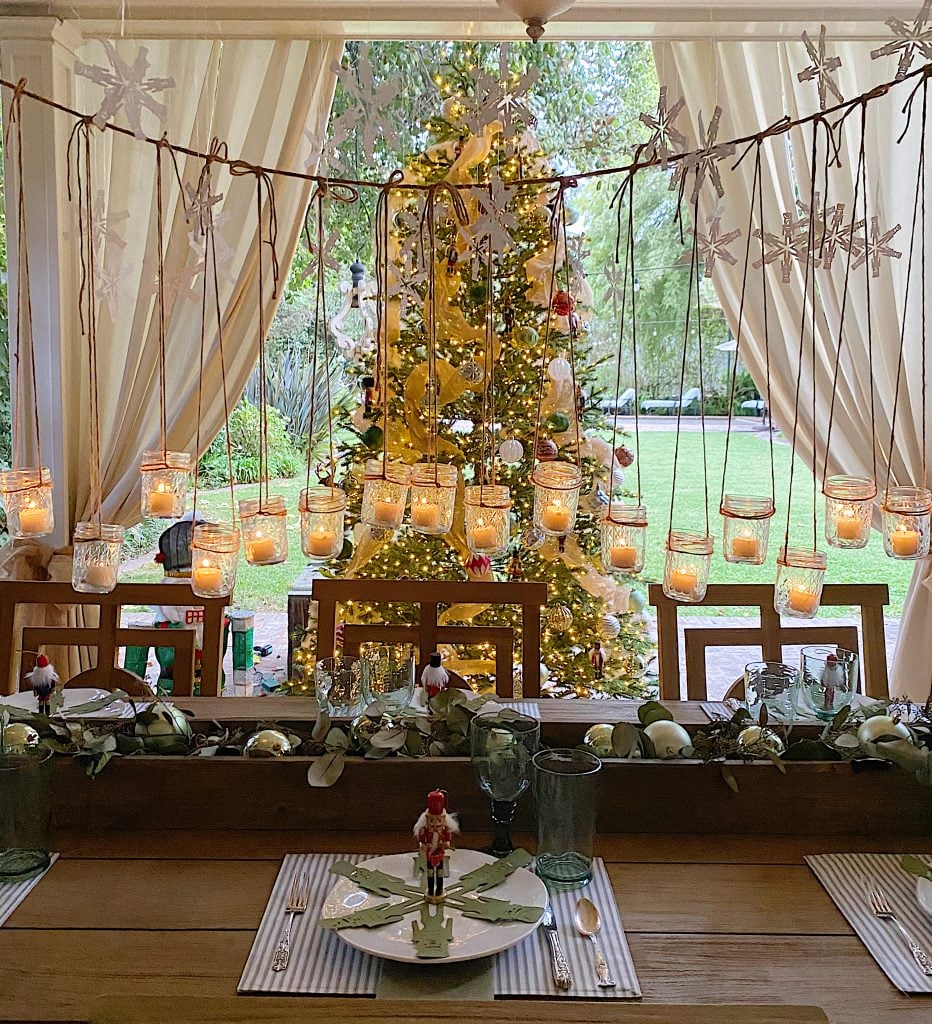This image captures a festive Christmas dining setup with an abundance of holiday decorations. At the center of the photo is a decorated Christmas tree adorned with white ribbons and green, red, and white ornaments, illuminated by simple white lights. The tree is placed in front of a window framed by white drawn curtains, through which daylight reveals a grass yard with green trees. The dining table, surrounded by brown square-framed chairs, features a snowflake placemat and a plate with a nutcracker, accompanied by silverware and an empty glass. A busy centerpiece brimming with Christmas ornaments runs along the length of the table. Hanging above the centerpiece, a twine clothesline supports mason jars wrapped with twine, each containing a lit tea light candle, adding a cozy ambiance to the scene. Garland and additional Christmas ornaments enhance the holiday atmosphere, making this an exceptionally detailed and festive display.